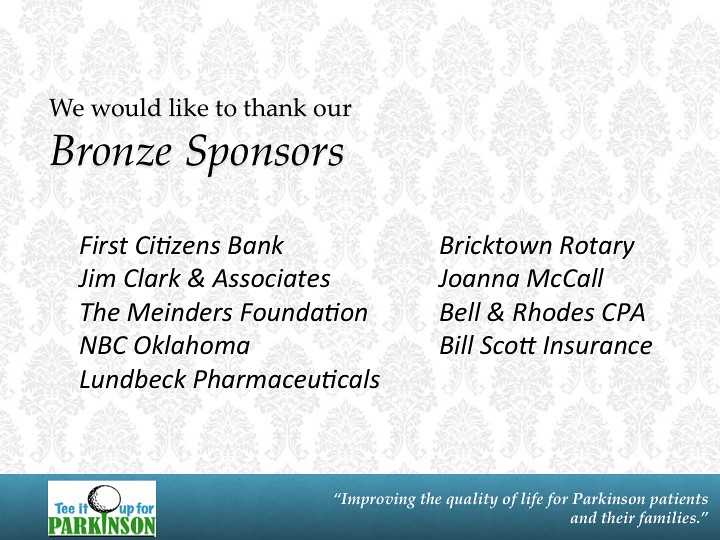**We Would Like to Thank Our Bronze Sponsors**

The top of the image prominently features the title "We Would Like to Thank Our Bronze Sponsors," with "Bronze Sponsors" in larger fonts. The central section is divided into two columns listing the sponsors' names in black text. The left column includes First Citizens Bank, Jim Clark & Associates, The Meanderers Foundation, NBC-Oklahoma, and Lumbag Pharmaceuticals. The right column lists Bricktown Rotary, Joanna McCall, Bell & Rhodes CPA, and Bill Scott Insurance.

The image has a background with subtle gray patterns on a white backdrop, enhancing the professional and formal tone. At the bottom, there is a blue horizontal bar. On the left side of this bar, a logo featuring a golf ball accompanies the text "Tee It Up for Parkinson’s," while the text on the right side reads, "improving the quality of life for Parkinson’s patients and their families." This phrase is set in quotations, emphasizing the mission of the event or campaign.